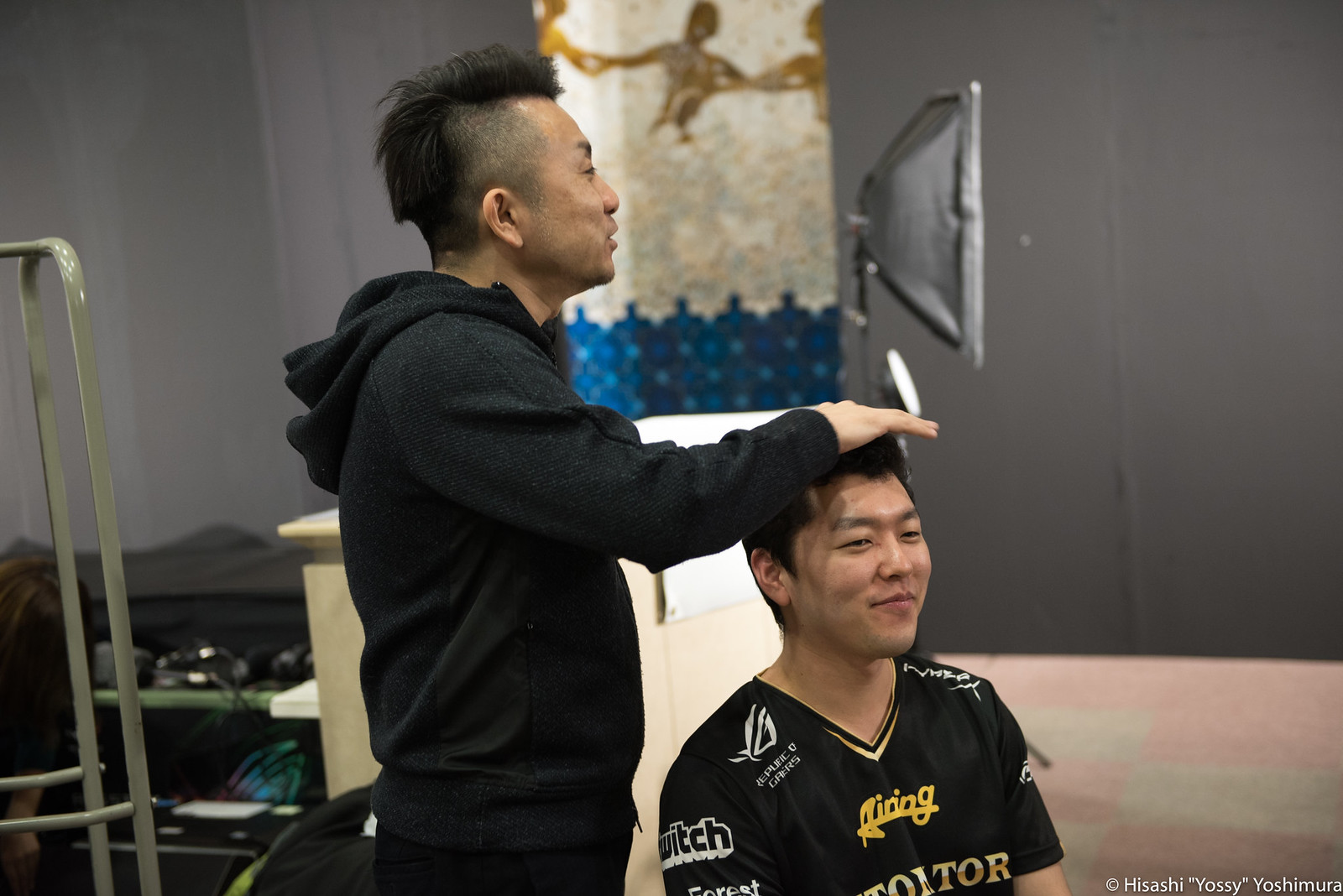This color photograph, captured by Hisashi Yoshimura, showcases two men, positioned centrally, in a landscape-oriented frame. The man on the right is seated, pictured from the chest up, wearing a dark eSports gaming jersey adorned with various brand logos such as the Republic of Gamers and Twitch. He has a slightly smug smile and looks off to the right. Standing to his left, another man, possibly a stylist or photographer, is engaged in conversation with someone out of the frame. This man sports long hair on top and back with shaved sides and wears a black hoodie. His right hand is extended over the seated man's head. The background is detailed with photographic equipment, including a light box on a tripod, speakers in the left corner, and a mural featuring a gold figure and blue patterns. The scene is set against gray walls and combines elements of photographic representational realism.